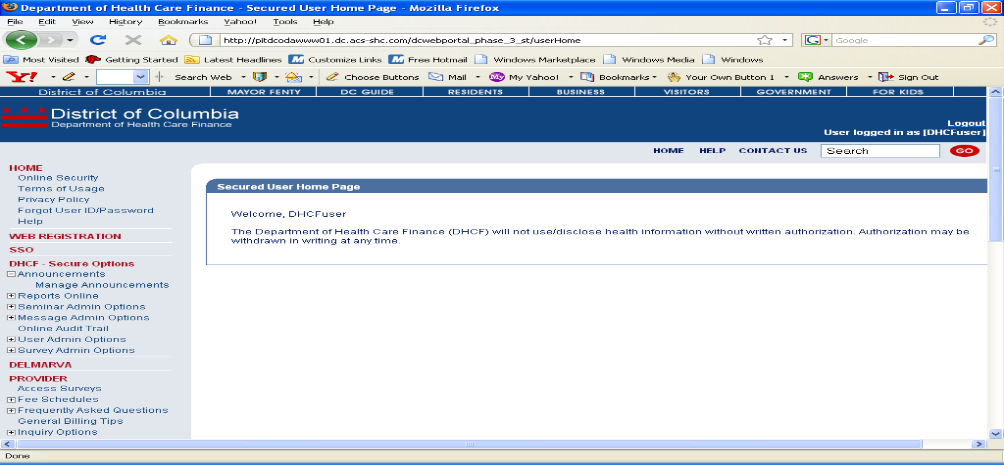This image displays a screenshot of a Firefox browser window open to the Department of Healthcare Finance's secured user homepage. At the top of the window, the blue title bar indicates "Department of Healthcare Finance - Secured User Homepage - Mozilla Firefox." Beneath this bar, typical browser menu options such as "File," "Edit," "View," "History," "Bookmarks," "Yahoo," "Tools," and "Help" are visible.

The address bar sits directly below the menu options, with several bookmarks lined up along the top. The main webpage content is from the District of Columbia's Department of Healthcare Finance. Prominently displayed is the title "District of Columbia Department of Healthcare Finance," along with additional headers referencing "District of Columbia Mayor Fenty," "DC Guide," "Residents," "Business," "Visitors," "Government," and "For Kids."

On the left side of the page, there’s a vertical navigation menu with options including "Home," "Web Registration," "SSO," "DHCF Secure Options," and "Delmarva Provider." To the right, a box titled "Secured Home User Homepage" welcomes the user with the message, "Welcome DHCF User."